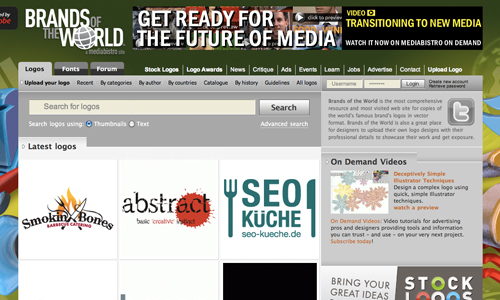A screenshot of a website showcases a dark green header at the top. On the top left corner, there's a logo for "Brands of the World" in white lettering. The word "Brands" is positioned on the top while "World" is at the bottom, with the 'O' in "World" featuring a light gray glow and a white grid. Adjacent to "World" is the word "THE" in all-caps gray text, and next to "Brands," "OF" appears in a similar gray text. 

To the right of the logo, there's an advertisement. The ad features a collage of photographs of people on the left, while on the right there is a black rectangle. Superimposed on the collage is large all-caps white text that reads, "GET READY FOR THE FUTURE OF MEDIA." On the black rectangle, the top-left part has yellow text in all-caps reading "VIDEO," with a yellow rectangle featuring a black circle to its right. Below this, larger yellow all-caps text reads, "TRANSITIONING TO NEW MEDIA." Following a line break, another line of all-caps text states, "WATCH IT NOW ON MEDIA BISTRO ON DEMAND."

Directly underneath this advertisement, there’s another header against the dark green background. On the left side, there are three tabs. The first tab is light gray with black text that says "LOGO." Next to it are two tabs that are half-medium gray on top and half-dark gray on the bottom, with white text reading "FONTS" and "FORUMS" respectively. To the right of these tabs, against the green background, is white text separated by thin vertical white lines.